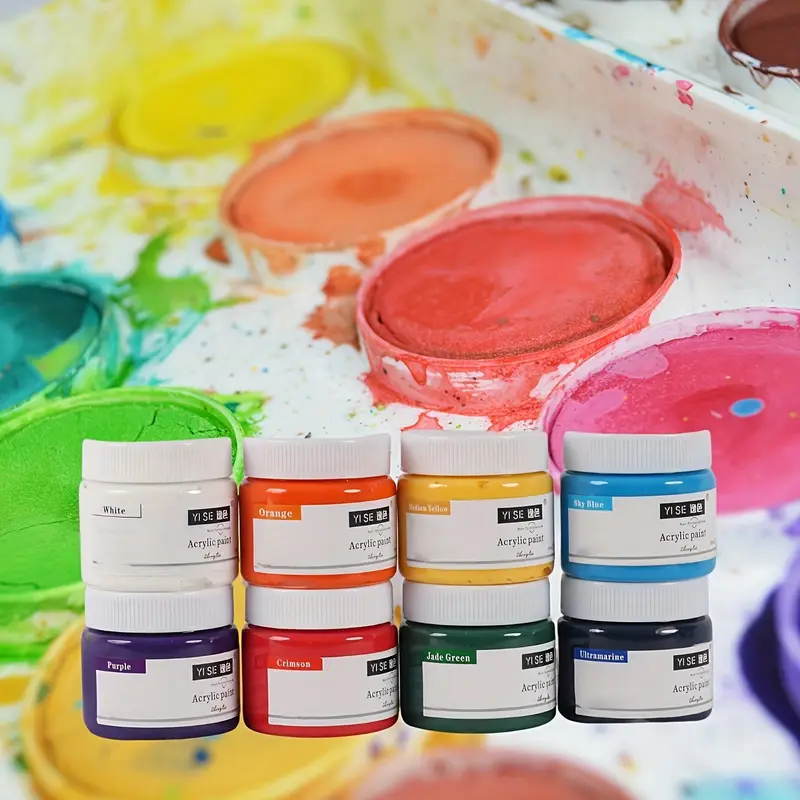This vibrant advertisement showcases a set of Yise Acrylic Paints in eight small plastic tubs neatly stacked in two layers. The set includes an array of colors: white, orange, yellow, sky blue, purple, crimson, jade green, and aquamarine, each labeled accordingly. The foreground containers are positioned against a backdrop of a well-used, colorful watercolor palette, evoking a sense of creativity and use. The background palette features a mix of colors—yellow, orange, red, pink, purple, aqua blue, lime green, and a deeper yellow—indicating the presence of a child's playful artistry, with dried and cracked paint wells adding a rustic, nostalgic touch. The superimposed product photo with its simple black and white Yise logos, including possible Chinese characters, contrasts with the chaotic, colorful background, making the image both eye-catching and joyful, ideal for inspiring budding artists.